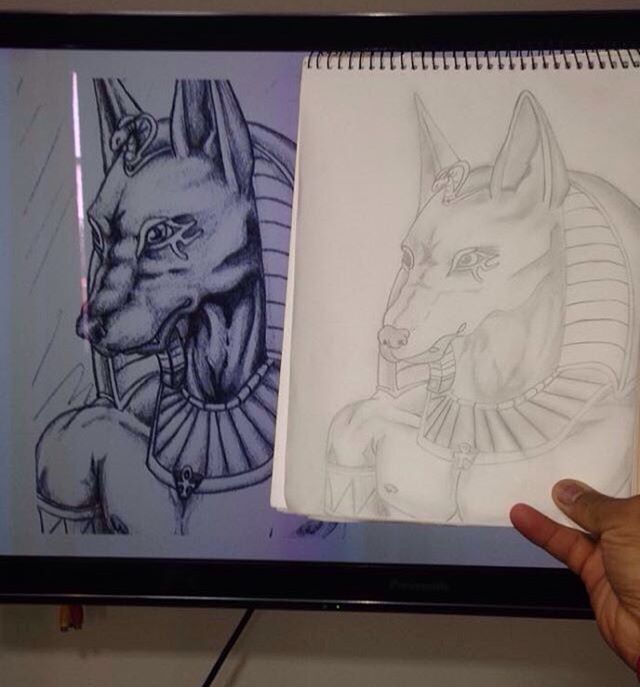This photograph captures a person holding a pencil sketch in front of a framed, high-contrast black-and-white drawing, both depicting an Egyptian-themed dog resembling the god Anubis. The Egyptian dog has long pointed ears, Egyptian-styled eyes with what appear to be tears, and a small snake emerging from between its ears. It is adorned with an elaborate headdress and folds of fabric reminiscent of pharaonic attire, complete with an intricate cross and armor around its chest. The framed original on the left, rich in detail, showcases the dog in a three-quarter profile facing left. The sketch, held by the person's right hand with their thumb and pinky visible, is drawn on a white paper with a dark spiral binding at the top and mirrors the overall design of the framed drawing, albeit with lighter shading and lower contrast, highlighting the artist's individual style differences.